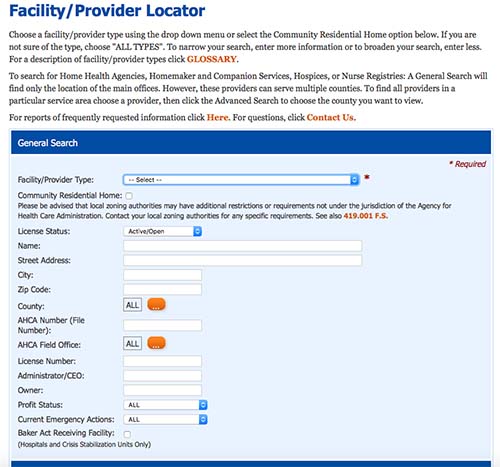**Detailed Caption:**

The image depicts an online interface for locating facilities and providers, labeled at the top as "Facility/Provider Locator." Users are prompted to select a facility or provider type from a drop-down menu or choose the "Community Residential Home" option. If uncertain about the type, users can opt for "All Types." To refine the search, more information can be entered, while less information will broaden the search. For explanations of the facility/provider types, a "Glossary" link is provided.

To search for specific types of providers such as home health agencies, homemaker and companion services, hospices, or nurse registries, a general search will only display the main office locations. However, these providers can serve multiple counties. For a comprehensive list of providers within a specific service area, users are advised to choose a provider and utilize the advanced search options to select the county they wish to view.

For frequently requested reports, a clickable link is available. For further inquiries, there is a "Contact Us" option. Below these instructions, a dark blue bar with white text reads "General Search." Beneath this bar, users can select a "Facility/Provider Type" using a drop-down arrow. There is an unchecked checkbox for choosing "Community Residential Home."

A cautionary note informs users that local zoning authorities might impose additional restrictions or requirements not governed by the Agency for Health Care Administration (AHCA), advising users to contact local zoning authorities for specific requirements, referenced as CSO 419.00 FS. 

Several search parameters are available, including "Resident Status" with options accessible via a drop-down arrow, and fields for entering "Name," "Street Address," "City," "Zip Code," "County," "AHCH Number," "File Number," "AHCA Field Office," "License Number," "Administrator/CEO," "Owner," "Profit Status," and "Current Emergency Actions." The option to select "Baker Act Receiving Facility" is presented with an unmarked checkbox, applicable only to hospitals and crisis stabilization units.